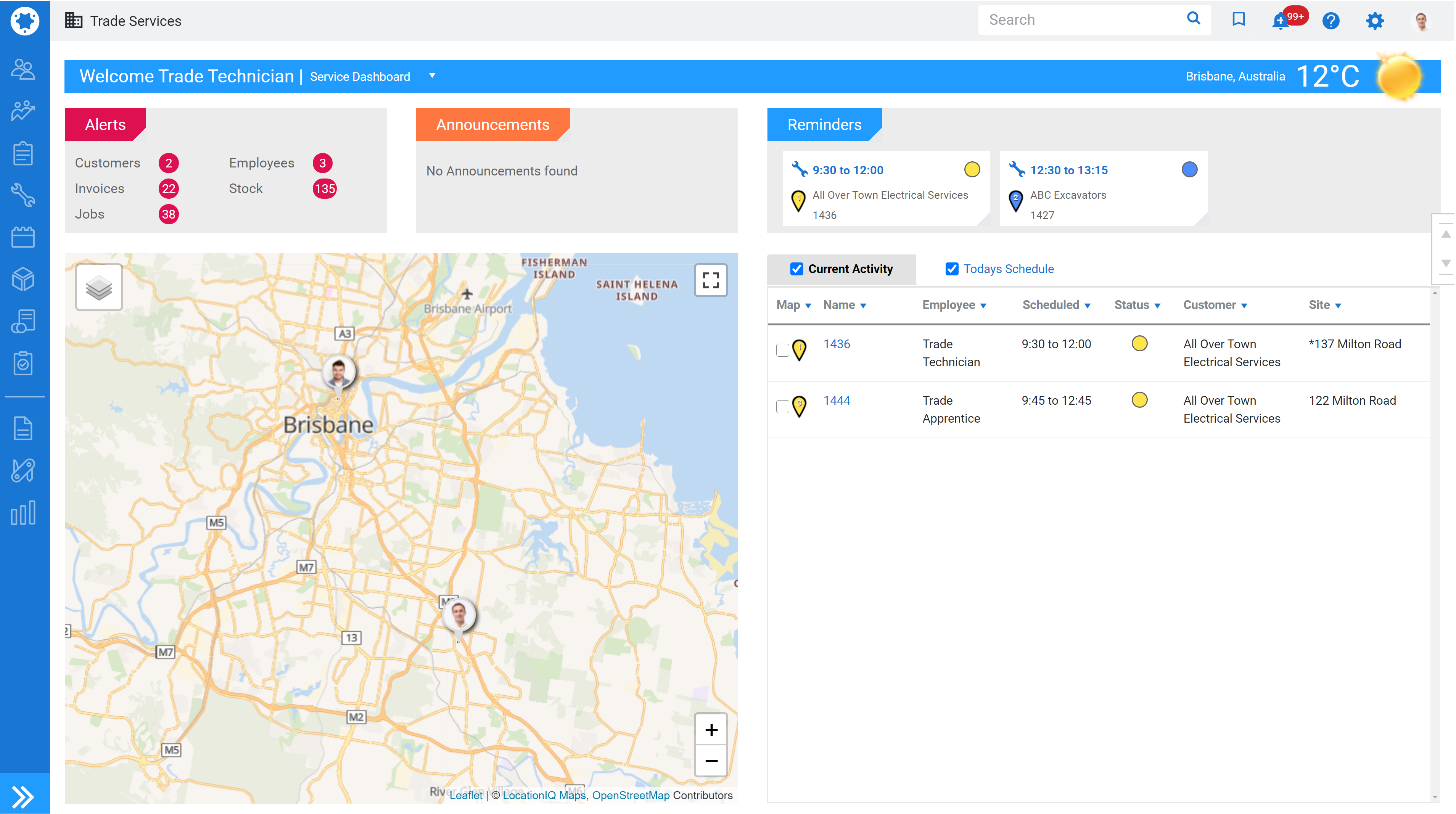Here is a cleaned-up and detailed caption for the image described:

---

The image depicts a webpage that features a map for locating services. On the left side of the interface, there is a vertical dark blue strip, approximately half an inch wide, featuring a circular icon with a blue star inside a six-sided star. Below this icon, there are eight clickable icons aligned vertically, followed by a separator line, and then three additional clickable icons. Each icon is outlined in white. At the bottom of this strip is a light blue square containing two right-facing greater-than signs.

Across the top of the webpage runs a narrow gray bar, also about half an inch in height. On the left side of this bar, it reads "Trade Services." On the right side, there is a search icon, a small blue square, and an alert icon highlighted by a red circle with a white ellipsis inside. This is followed by a blue circle containing a white question mark, then a settings icon, and a lock icon.

Below this gray bar, there is a narrow white border, under which a blue section with white text welcomes the user with "Welcome Trade Technician." Beneath this, it mentions "Service Dashboard." On the right side of this area, the weather is displayed with a sun icon and the text "12 degrees Celsius" indicating the temperature in Brisbane, Australia.

Further down, the left side of the page features a light gray rectangle titled "Alerts" in its top-left corner, listing five items each accompanied by a red circle with a white number inside. Adjacent to this, there's a light blue rectangle labeled "Announcements," marked by an orange tab; it notes "No announcements" underneath the label.

The main section of the page displays a map extending to the bottom. The map shows blue for water in the top-right corner and a mix of tan and green for land, with yellow lines denoting roads. At the center of the map is a profile picture labeled "Brisbane."

On the right side of the webpage is a lengthy rectangle. The top-left corner of this rectangle is labeled "Reminders." Below this, there are two white squares with reminder items. Following these reminders is a section labeled "Current Activity" on the left side, and "Today's Schedule" to the right. The "Current Activity" section includes a gray bar at the top, and details listed below about the user's current activities and today's schedule.

---